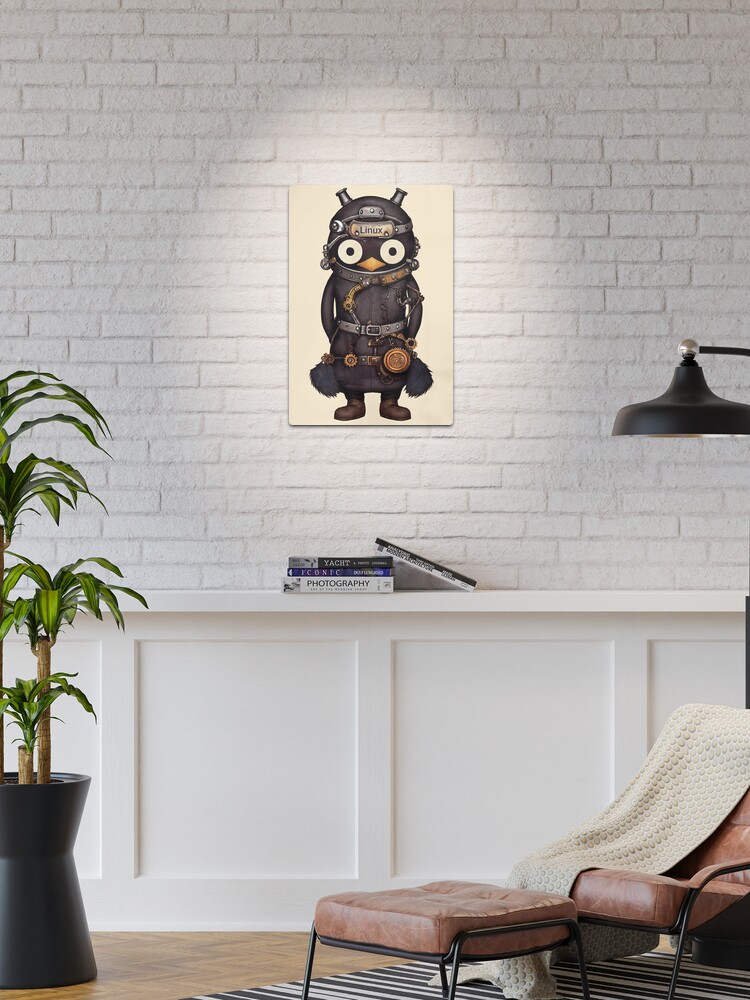The image depicts a minimalistic studio space featuring a meticulously designed wall adorned with an art piece. The wall is predominantly white brick, accented with a wooden backing on the lower half. Central to this setting is a medium-sized artwork illuminated by a spotlight, showcasing a cartoonish penguin dressed in pilot gear, complete with a helmet, boots, a belt, and a diamond-shaped yellow beak. The word "Linux" is prominently displayed on the piece, hinting at its thematic inspiration. Below the artwork, a white shelf holds an array of books titled "Photography," "Iconic," and one referencing yachts. To the left of the artwork stands a black pot housing a plant with gray, green, and brown hues. Adjacent is a brown leather chair draped in a creamy white throw, accompanied by a matching footrest. A black lamp adds a subtle element of contrast to the predominantly light and airy color scheme. The room exudes a contemporary and clean aesthetic, blending simplicity with carefully chosen decor to create a serene and inviting atmosphere.